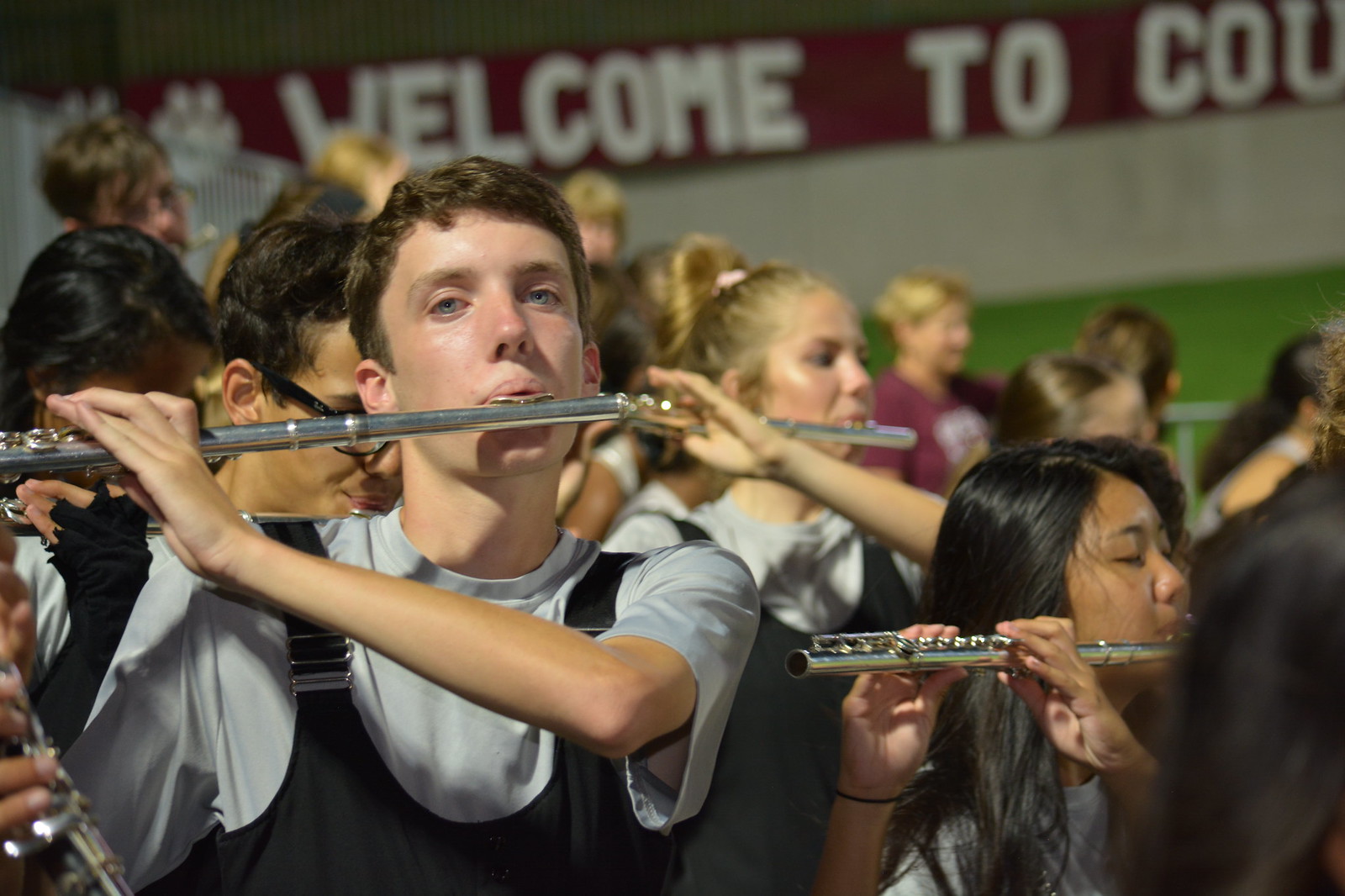In an indoor or possibly outdoor setting at a football stadium, a photograph captures a section of a marching band, focusing on the flute players. Prominently in the foreground is a young white boy with short brown hair, wearing black suspenders over a light gray short-sleeved shirt. He occupies a significant portion of the image, with his flute raised to his mouth, his hands positioned on the keys, and his gaze directed generally towards the camera, though not directly at it. To his right stands a shorter Asian woman, her black hair parted in the middle, also playing the flute with her eyes partly closed. She wears a black wristband on her right wrist. Behind them is a blonde woman with her hair tied back, similarly dressed in black overall-like attire over an off-white shirt, matching the boy’s outfit. In the background, there is a man with dark hair and black-framed glasses, leaning slightly forward, and several blonde women. The stadium’s stands show some spectators, including one wearing red. A partially blurred sign in the background reads, "Welcome to COL," set against a maroon background. The grassy field can also be seen behind the band.